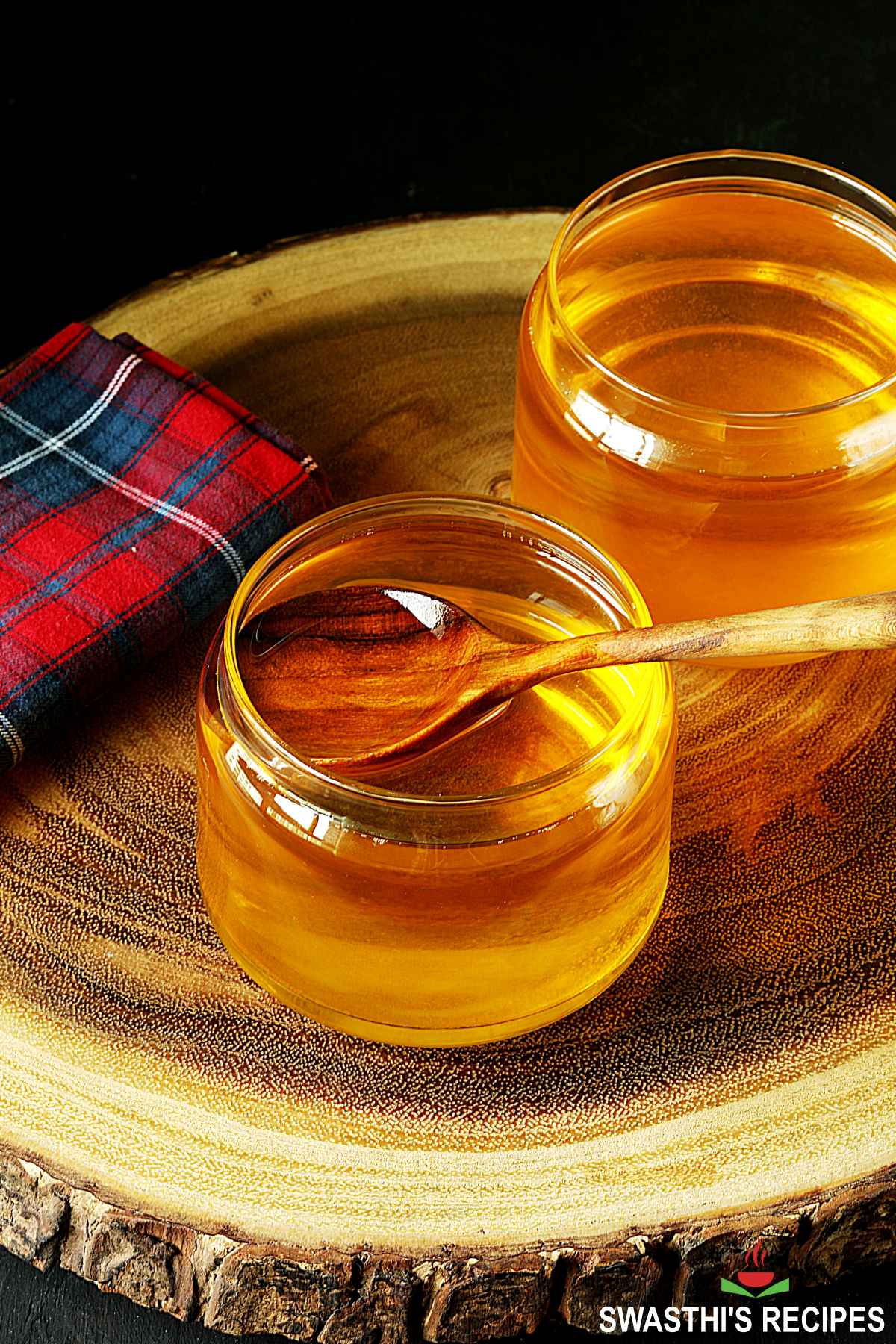The photograph depicts two small, gold-hued jars of honey placed on a rustic wooden slab, reminiscent of a tree trunk slice, used as a serving platter. The front jar features a medium-sized spoon with a wooden handle. To the left of the jars, there is a neatly folded plaid napkin, characterized by its red, blue, and white pattern. The background contrasts starkly with the setup, being completely black, which highlights the honey jars and napkin. At the bottom right corner of the image, white text reads "Swasthi's Recipes," spelled S-W-A-S-T-H-I-apostrophe-S, accompanied by a logo above: two light green lines resembling an abstract book with a red heart situated in the center.